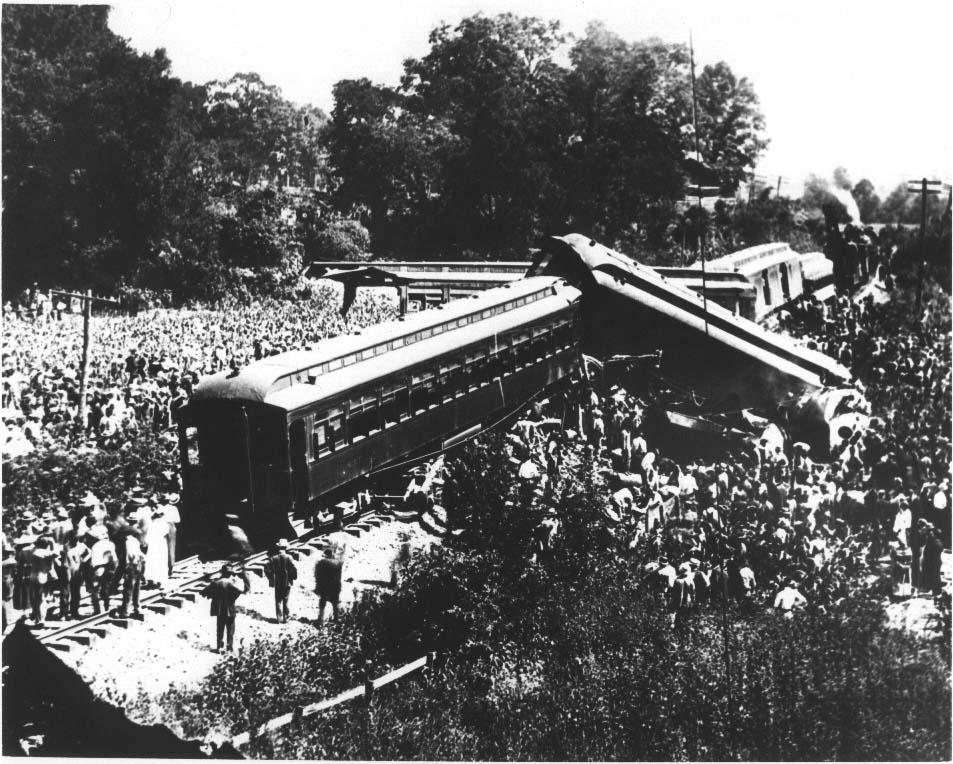This old black-and-white photograph, likely from an early 20th-century train accident, depicts a severe collision where two passenger train cars have derailed and lie diagonally across one another, forming an X shape. The image is horizontally oriented and approximately six inches wide by five inches tall. In the scene, a large group of people, many wearing hats, are standing on both sides of the train tracks, possibly involved in rescue efforts. The background is lined with tall trees, light poles, and a white sky, indicating a daytime setting. The wreckage appears quite severe, with train cars piled atop each other and fields of brush visible in the lower corners of the photo. Despite the apparent intensity of the crash, no casualties are visible, suggesting the photo may have been taken post-rescue. The rectangular photograph captures the chaotic aftermath of the crash with a crowd of onlookers taking in the tragic scene.